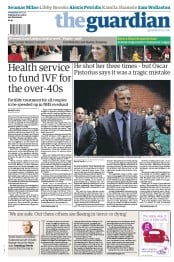The image features a prominently displayed article from The Guardian newspaper. The headline reads, "Oscar Pistorius shot her three times, claims it was a tragic mistake." The photograph accompanying the article captures Oscar Pistorius in a suit jacket, surrounded by people in a courtroom setting. The article beneath the headline delves into the details of the incident but appears too blurred to read clearly. 

Adjacent to this main article on the left, another headline discusses a health service initiative, stating, "Health service to fund IVF for women over 40." Beneath this headline, a byline with the author's name, the publication date, and time can be observed, although specifics are illegible due to blurring.

The newspaper's masthead is prominently displayed at the top, with "The Guardian" in a darker blue font against a sky-blue background. To the left of the masthead is a barcode, and above it, a header intended to capture readers' attention with sensationalized snippets. Below the barcode are three small images, with only the middle one being distinguishable; it appears to show Kate Middleton, presumably accompanied by an article related to her and Prince William. Each image is topped by its own brief headline.